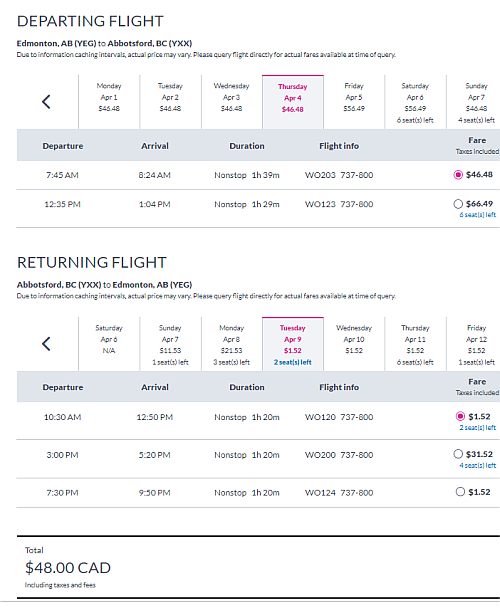**Image Caption:**

The background is divided into white at the bottom and black in the upper left-hand corner. In this upper section, it reads "Department of Flight, Edmonton, AB (YEG2) - Abbotsford, BC (YXX)." A note appears, stating, "Due to information catching intervals, actual prices may vary. Please query flight directly for actual fees available at the time of querying." An apple symbol pointing to the left is included.

The flight prices and availability are listed as follows:
- Monday, April 1st: $45.48 (text slightly blurry)
- Tuesday, April 2nd: $46.48
- Wednesday, April 3rd: $46.48
- Thursday, April 4th: $46.48 (highlighted in magenta)
- Friday, April 5th: $56.49
- Saturday, April 6th: $56.49 (six seats left)
- Sunday, April 7th: $46.48 (four seats left)

A black-green border runs across the image, with the text in black reading: "Departure, Arrival, Duration of Flight, Info, Fare (TOEX is included)."

The details for specific flights are listed as follows:
- 7:45 AM to 8:24 AM, non-stop, 1H39M, Flight W0203, 737-800 (highlighted in magenta with a fare of $46.48)
- A thin gray line divides this from the next entry:
- 12:35 PM to 1:04 PM, non-stop, 1H29M, Flight W0123, 737-800 (outlined circle with a fare of $66.49 and "six seats left" in blue)

Below, in black text, it says "Return Flight," and then reads "Abbotsford.com, ABC (YXX) - AB (YEG)."